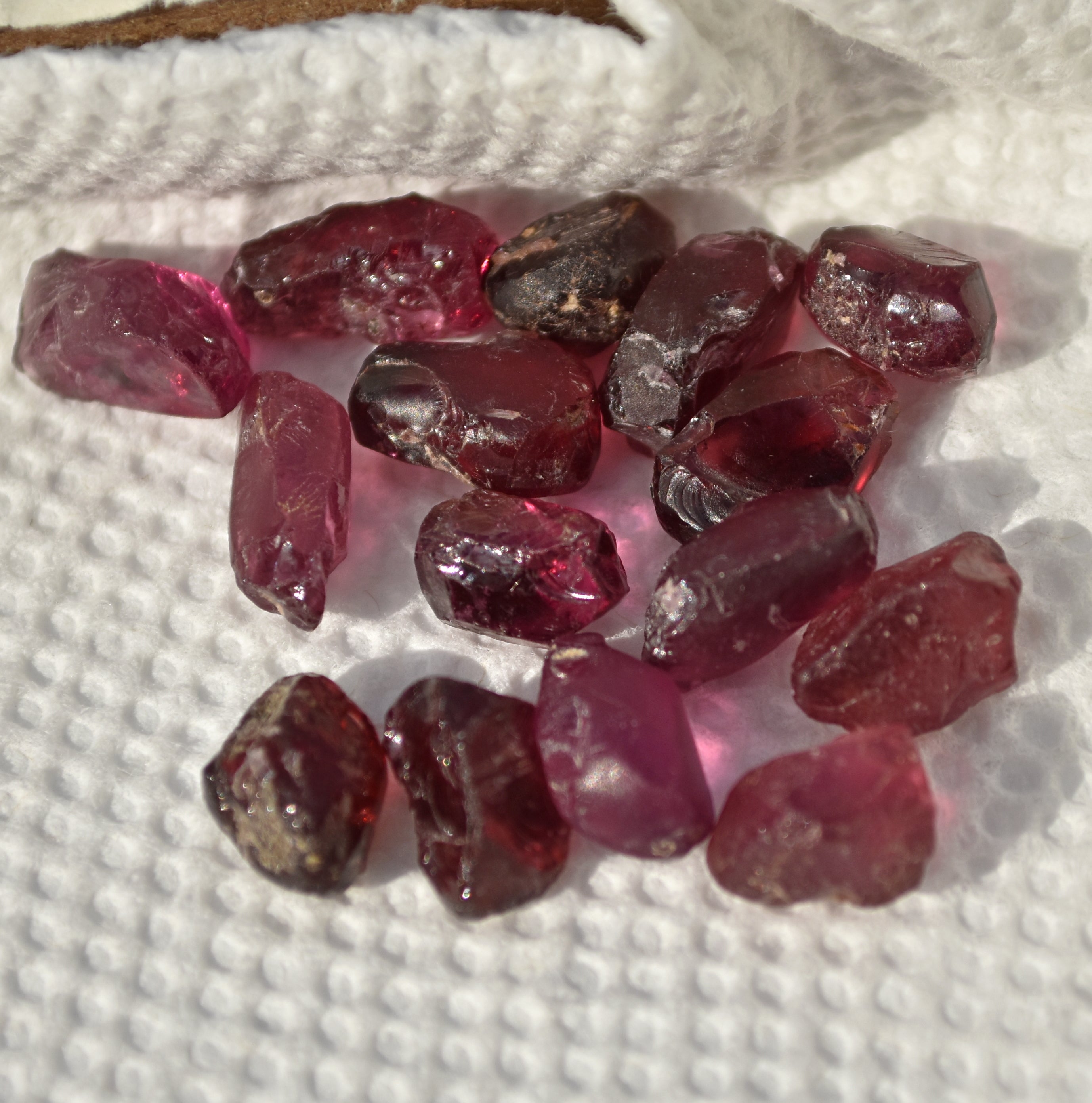The image depicts a close-up view of several small, irregularly shaped stones or gems, which are red to dark red, some almost black in color. These stones, potentially gemstones or melted material, are clustered together on a white paper towel that serves as the background. The white fabric has a light egg crate pattern. There are approximately 12 to 15 stones in total, varying in shades from a light reddish-pink to a dark, ruby red, with one particularly dark stone that looks almost black. Some also have visible dirt and are rough-cut rather than uniformly shaped. The stones cast distinct shadows to their right, suggesting that the light source is positioned to the left. The overall image is bright and zoomed in, making the minute details of the stones and their shadows clearly visible, particularly the rocks in the rear that are more in focus compared to the slightly blurry ones in the foreground.